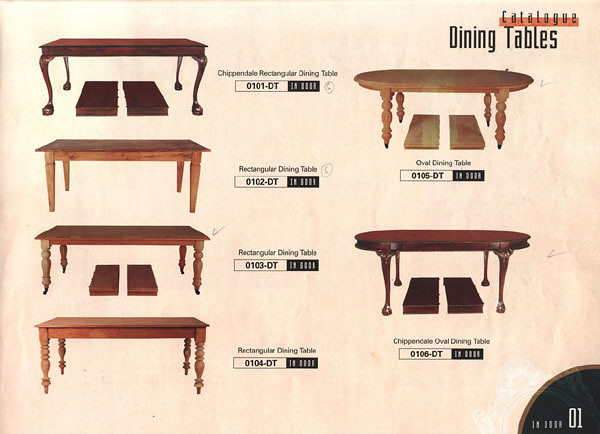The image is a catalog page displaying six different styles of dining tables. The top right corner of the page reads "Catalog Dining Tables." On the left column, the top-left table is labeled "Chippendale Rectangular Dining Table," distinguished by its ornate design and dark redwood material. Below it are three other tables, each simply labeled "Rectangular Dining Table," featuring varying designs on the legs, ranging from simpler to more ornate styles. On the right column, the top-right table is labeled "Oval Dining Table," with an oval tabletop and ornate legs. Below it is another dark, rounded table labeled "Chippendale Oval Dining Table," similar in material and design to the Chippendale table on the top left. The bottom right-hand corner includes a design marked "Indoor 01," and the overall page has an off-white background.